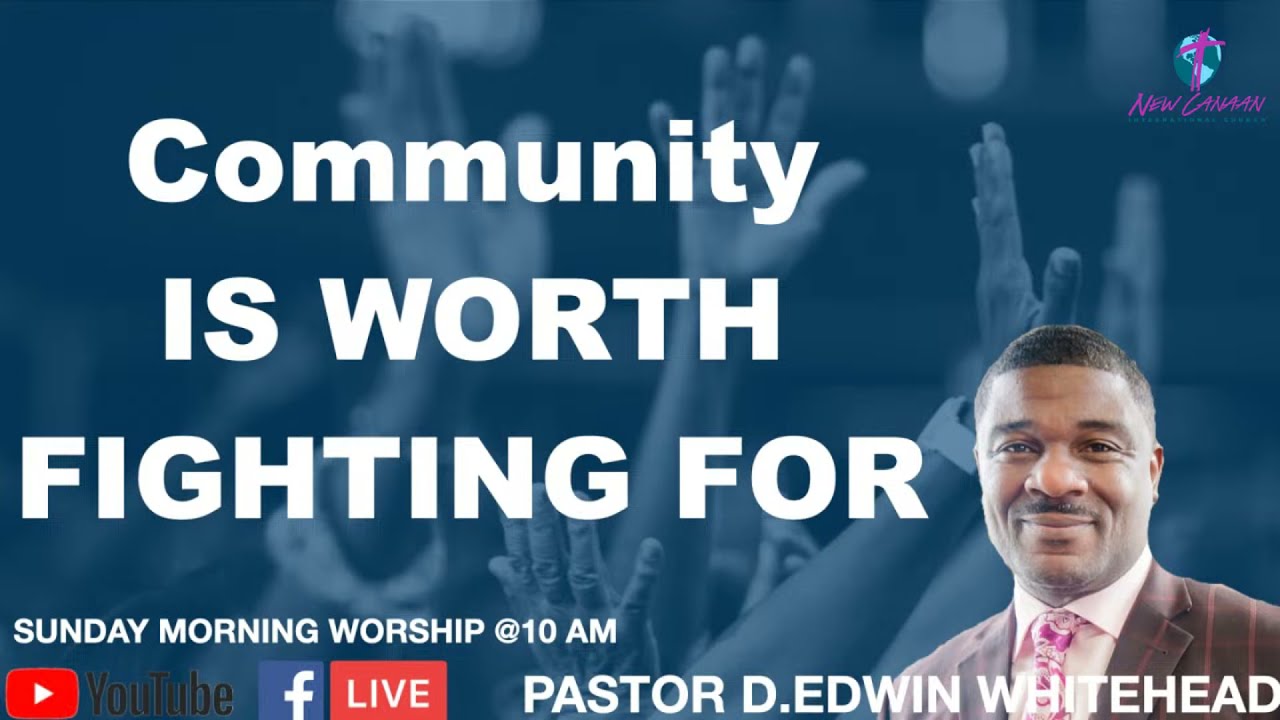The image features an advertisement for a Sunday morning worship service at 10 a.m., prominently displaying the text "Community is Worth Fighting For." The scene includes a blue background with a subtle overlay of blurred hands raised in worship, adding a sense of community and participation. In the top right corner, there is a church logo—a globe with a purple cross—accompanied by the text "New Canaan." The bottom left corner highlights the YouTube and Facebook Live logos, indicating where the service will be broadcast. On the bottom right is a headshot of Pastor D. Edwin Whitehead, a black man with short black hair, a mustache, and dimples, wearing a brown pinstripe suit, a light pink shirt, and a floral pink and white tie. His name appears beneath his image in white text. The overall composition and color scheme convey a welcoming and professional atmosphere suitable for a church service announcement.